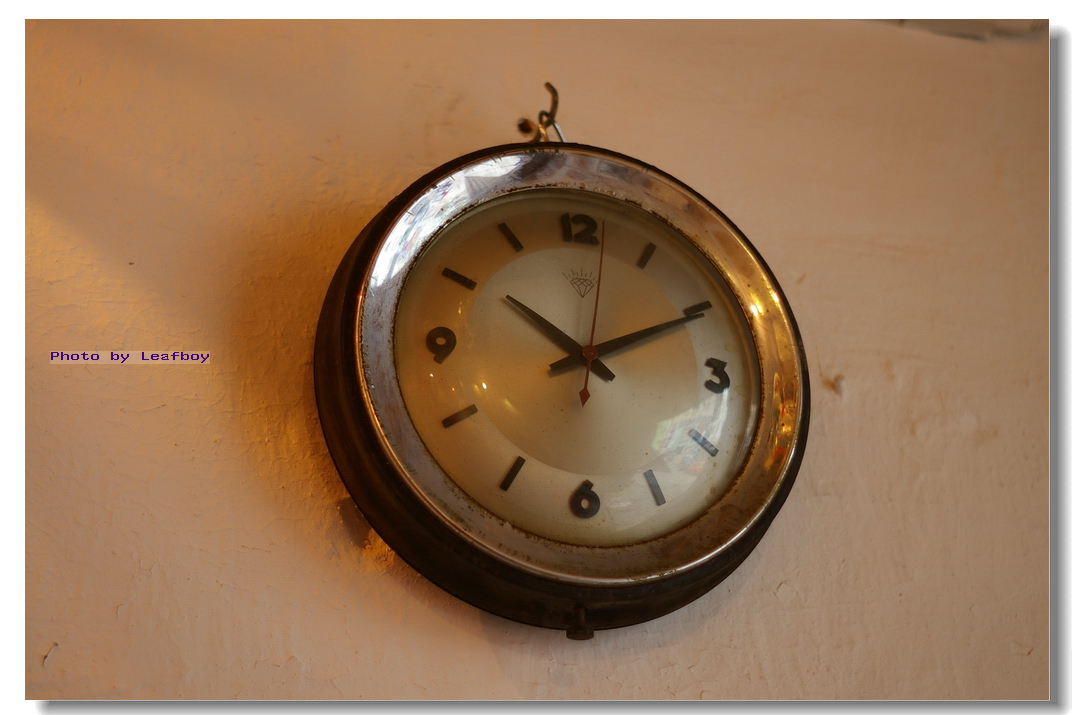This photo captures a vintage, all-metal wall clock characterized by its rusted appearance and unique design. The clock is mounted on a stark white wall with peeling paint, creating a contrast that highlights its antiquated charm. The numbers 12, 3, 6, and 9 are distinctly marked, while simple lines indicate the other hours. A peculiar spring is attached to the top of the clock, adding an unusual element to its structure. The time displayed is 10:11, and both minute and second hands are visible beneath a glass front. On the far left side of the image, a label reads "Photo by Leaf OALEAFOY." The clock is prominently centered in the photograph, making it the focal point.